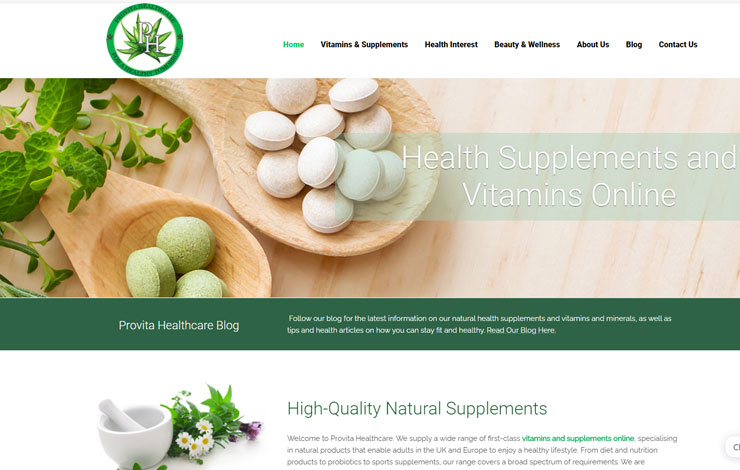The image displays a web page with a long rectangular layout, focusing on health supplements and vitamins available online. At the top, there is a green circular icon featuring an illustration of herbs. The navigation bar includes links to Home, Vitamins and Supplements, Health Interest, Duty and Wellness, About Us, Blog, and Contact Us.

The main image showcases a light blonde wood counter with two wooden spoons. The larger spoon holds white tablets, while the smaller one contains green tablets. Next to the spoons are some green herbs.

At the bottom of the image, there is a darker green banner that reads, "ProVita Healthcare Blog. Follow our blog for the latest information on our natural health supplements and vitamins and minerals, as well as tips and health articles on how you can stay fit and healthy. Read our blog here." This section includes an icon of a pestle and mortar, along with images of flowers.

Following this, the text introduces ProVita Healthcare: "High Quality Natural Supplements. Welcome to ProVita Healthcare. We supply a wide range of first-class vitamins and supplements online, specializing in natural products that enable adults in the UK and Europe to enjoy a healthy lifestyle. From diet and nutrition products to probiotics to sports supplements, our range covers a broad spectrum of requirements. We are..." The text cuts off at this point.